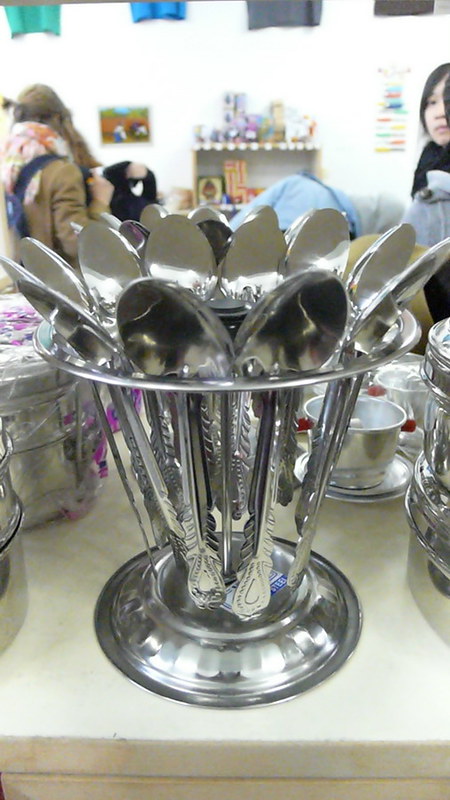The image depicts a bustling storefront, featuring a neatly organized display on a white countertop. The focal point is a silver canister holding an assortment of silver spoons. The canister itself is clear with a rounded base, ornate with a silver wire running through the middle to support a silver-toned cup at the top, which is secured with a black rubber stopper. Each spoon is meticulously arranged with the handles pointing downward and the spoon heads facing upward, radiating from the center of the canister. Surrounding the main display, additional silverware items can be seen on both the right and left. In the background, a few shoppers with backpacks peruse the store, adding a lively atmosphere to the scene.